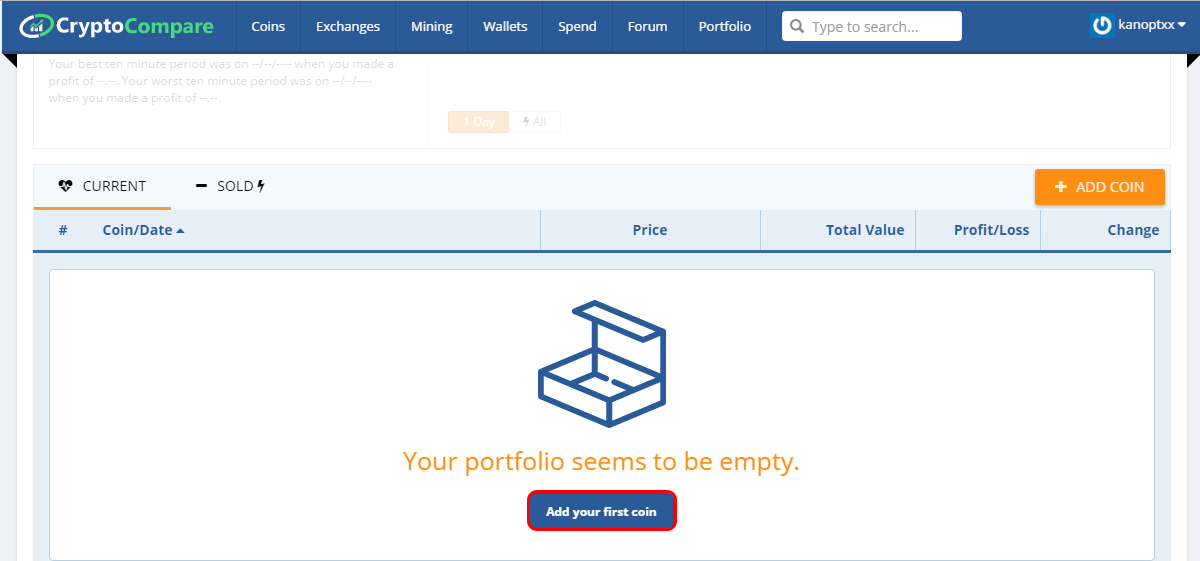The image depicts the interface of a cryptocurrency comparison website. At the top 10% of the screen, there is a prominent blue banner displaying "Crypto Compare" in white and green text. To the left of the banner text, there is an oval graphic that is half white and half green. To the right of the banner text are several navigational options in white: "Coins," "Exchanges," "Mining," "Wallet," "Spend," "Form," and "Portfolio." Adjacent to these options, there is a white search box with a gray magnifying glass icon inside, accompanied by the placeholder text "Type to search." To the right of the search box, a blue power button icon with a white power symbol is visible, followed by a dropdown menu labeled "Cannot TXX."

Below this navigation bar, a section with a white background features a "Current" tab highlighted in orange, which includes a heartbeat icon. Next to "Current," there is another tab labeled "Sold," represented by a lightning bolt icon, all in black text. To the right of these tabs, an orange button with white text and a plus sign reads "Add Coin."

Underneath the "Current" tab, there is a light blue header row with darker blue text listing columns: "№/Coin/Date," "Price," "Total Value," "Profit/Loss," and "Change," all denoted with an upward arrow indicating sortable columns.

The main content area displays a clipart image of a cardboard box with a blue outline and white interior. Below the image, a message in orange text reads, "Your portfolio seems to be empty." At the bottom of this section, a blue box with a red outline invites users to "Add your first coin," written in white text.